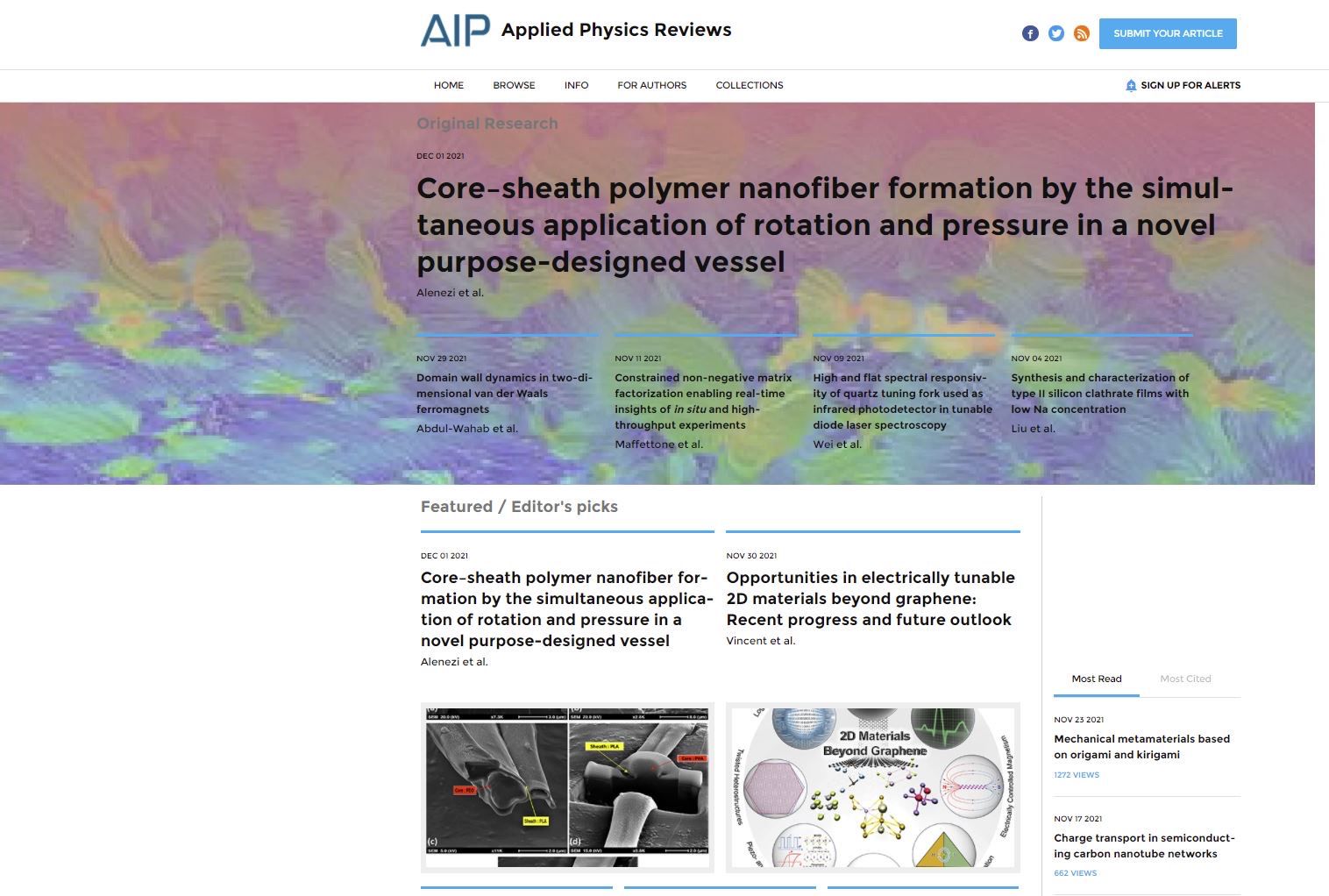This detailed image showcases a webpage from the journal "Applied Physics Reviews," specifically featuring an article titled "Core-Sheath Polymer Nanofiber Formation by the Simultaneous Application of Rotation and Pressure in a Novel Purpose-Designed Vessel." Prominently displayed at the top right are options for submitting an article, and icons linking to social media platforms such as Facebook and Twitter. Additionally, a link for signing up for alerts is available. The page's categories, arranged neatly in a navigation bar, include Home, Browse, Info for Authors, Collections, Original Research, and the specific publication date of December 1, 2021.